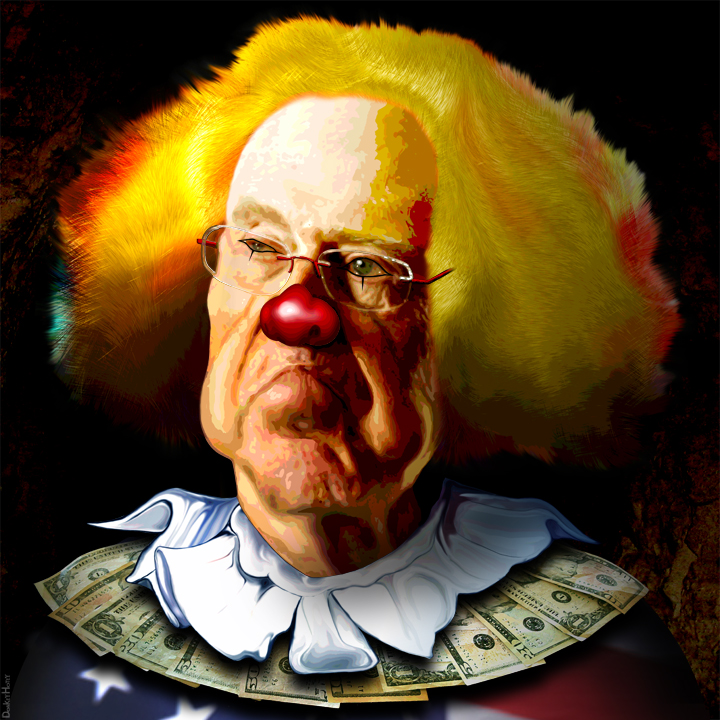The image is a detailed painting of a melancholic clown. At the center of the composition is a light-skinned man characterized by his saggy, wrinkled, and frowning face that is notably marked by droopy cheeks. His bald head is adorned with a voluminous yellow, red, and orange wig styled to hang to the sides, rather than up. The clown wears thin, rimless wire glasses, and one of his eyes is open while the other is partially shut, accentuated by thin black tear marks typical of clown face paint. A prominent red, fake clown nose sits at the center of his face. Beneath his face, he sports a large, ruffled white collar. Cascading below this collar is another, made of various U.S. dollar bills in denominations of $1, $5, $10, $20, and $50, fanned out underneath. At the bottom left of the image, a portion of the American flag can be discerned, featuring its blue field with white stars, while on the bottom right, parts of red and white stripes are visible, though mostly cropped out. The background of the painting features a mix of dark tones, including black, with hints of rust red and yellow particularly visible at the top left and bottom right corners. This dark backdrop creates a stark contrast to the bright and detailed foreground, emphasizing the somber and poignant nature of the clown's depiction.